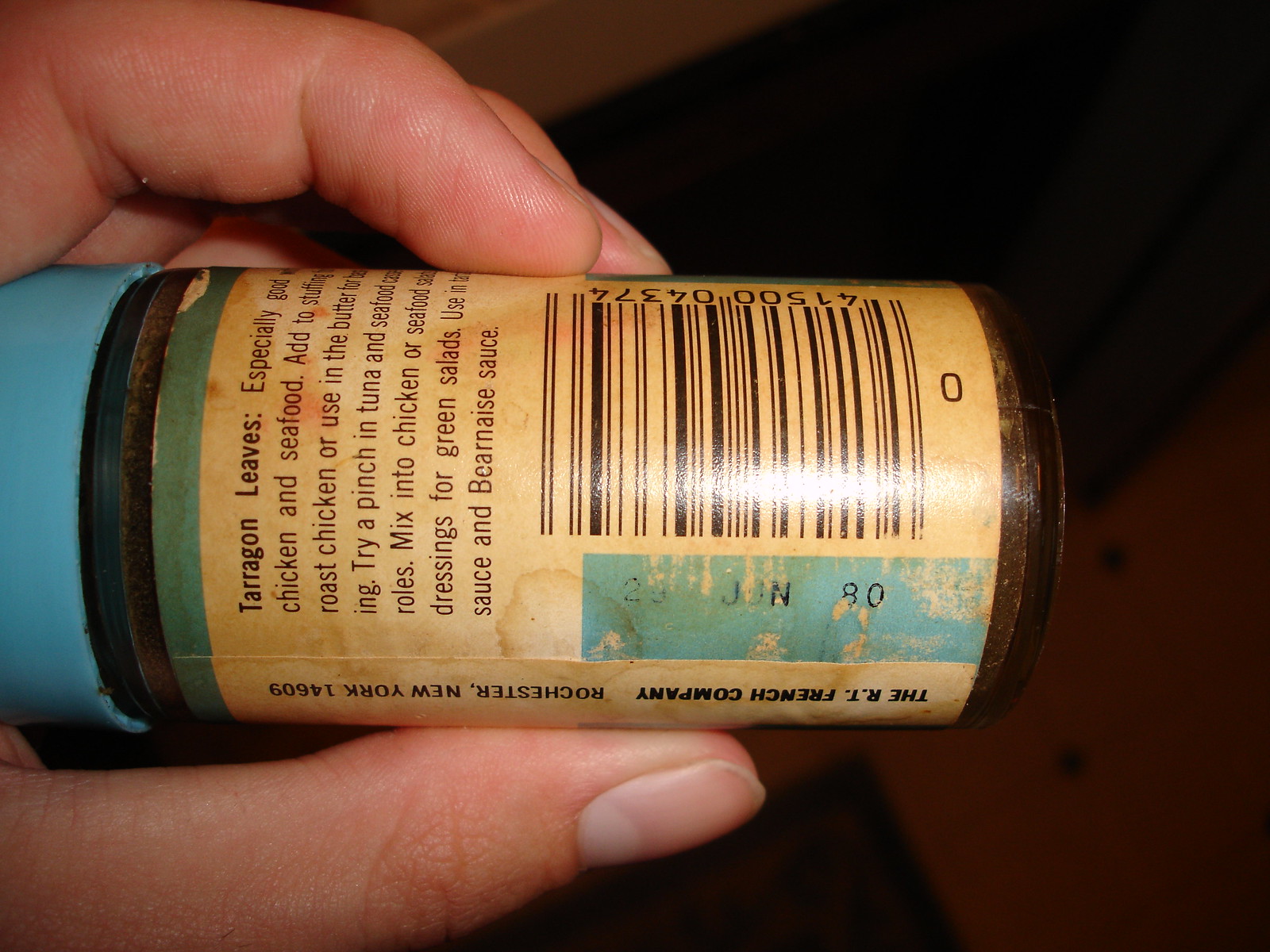The image depicts a first-person point of view of an individual with a fair complexion holding an aged spice bottle in their partially visible left hand against a brown background. The bottle, held sideways with the thumb underneath and fingers on top, features a tan label that has likely darkened over time and a blue lid. The label prominently displays "Tarragon Leaves" and provides extensive usage suggestions, including adding to chicken and seafood dishes, stuffing, roast chicken, butter, tuna and seafood casseroles, chicken or seafood salads, green salad dressings, and béarnaise sauce. Some instructions on the label curve out of view due to the bottle's shape. Additionally, the label includes a barcode, and on the side, it is marked with "The R.T. French Company, Rochester, New York 14609." Notably, there is a blue label that indicates the date "June of 90," suggesting the tarragon leaves are quite old.